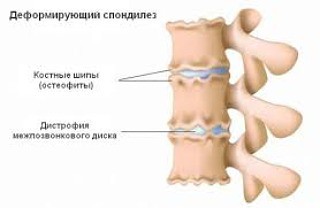The image is a detailed graphic depiction of three vertebrae of the spine, along with additional segments of the spine, presented on a white background. These vertebrae are illustrated in a light pinkish or beige color, with the intervertebral discs shown in a light blue, cylindrical shape. Black text is used for labeling various parts, with lines indicating specific anatomical features. The labels, written in Russian, include a bold title in the upper left corner and several lines of text to the left providing further annotations. This detailed spine graphic clearly aims to anatomically identify and explain parts of the vertebrae and discs.